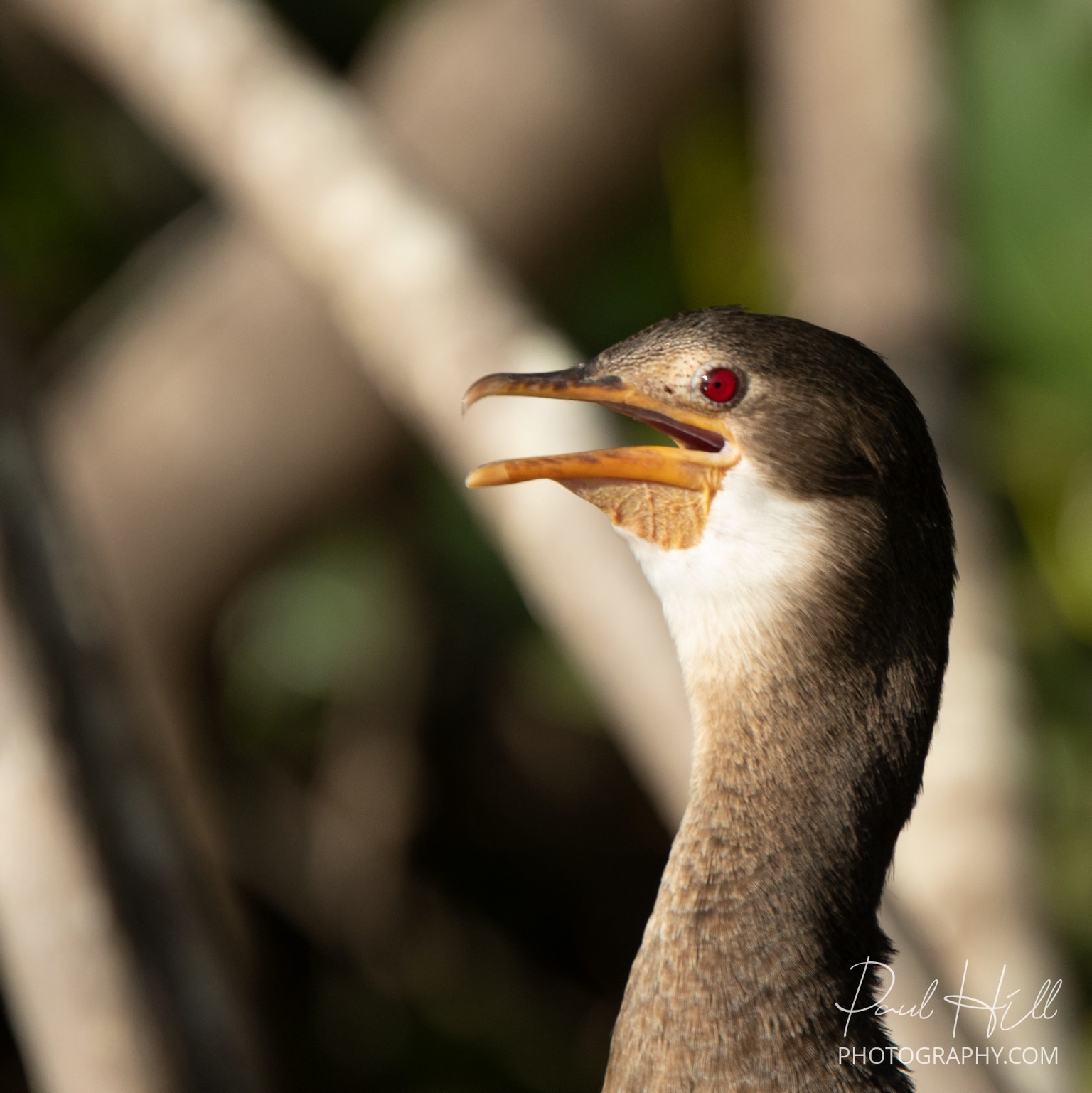This is a detailed close-up image of a bird, specifically a cormorant, known for its prevalence in the southern states of America and warmer tropics. The bird, positioned on the right-hand side of the image, is showcased in profile with its beak open, looking towards the left. It features striking red eyes and a pointy top beak that is yellowish-orange with black markings. The bird's plumage includes dark brown feathers, with lighter shades transitioning to white around the neck and face. The background is a heavily blurred depiction of trees and grass, providing a sense of a forested area. A signature in fancy white lettering reading "Paul Hill" and the text "photography.com" are positioned in the bottom right corner. The dominant colors in the image are shades of brown, gray, white, and green, which blend harmoniously to highlight the focus on the bird. There are no other animals, people, or additional text present in this photograph.